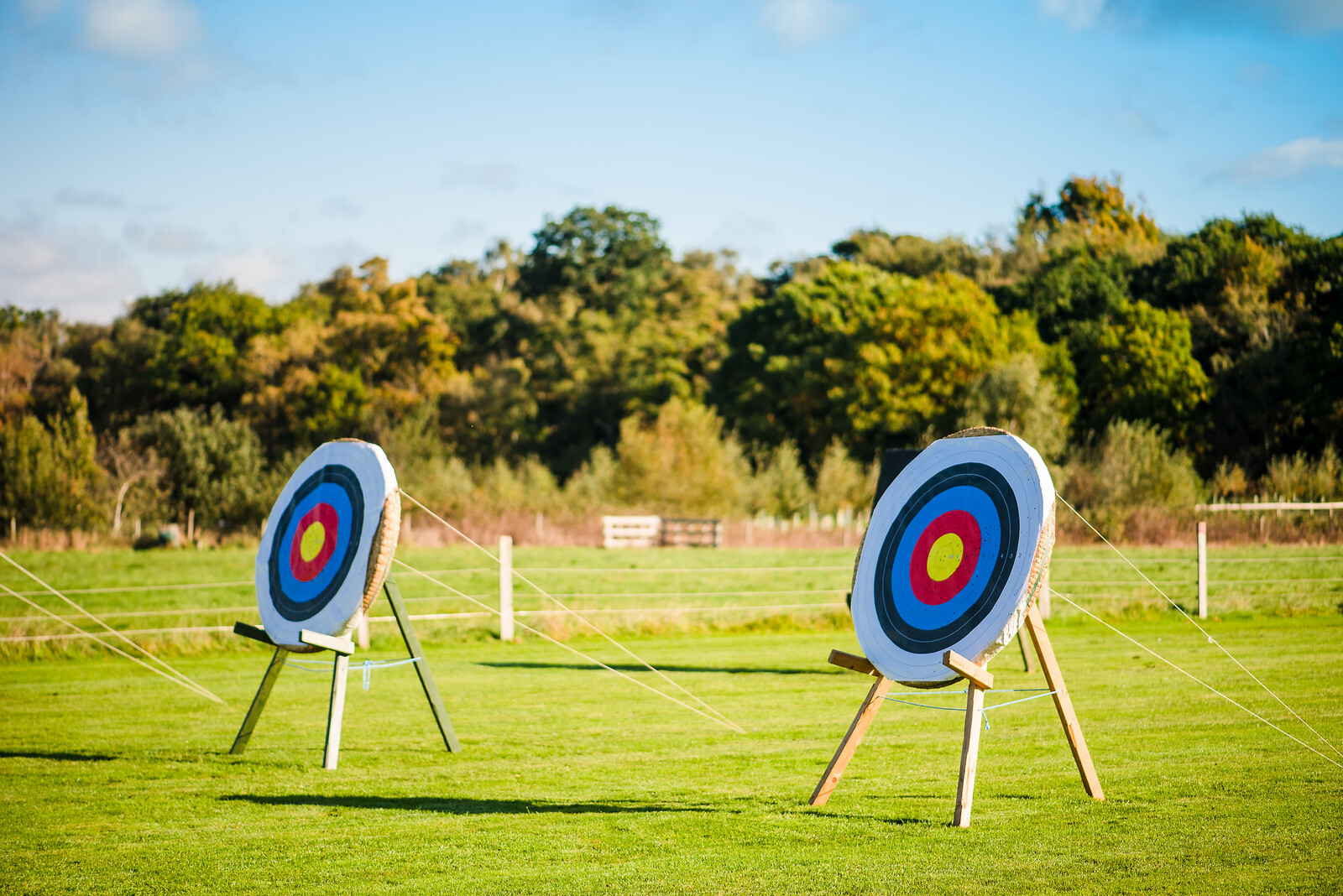This is a detailed color photograph of a target range set in a well-maintained, mowed field surrounded by a heavily forested area. The image prominently features two large archery targets positioned on rudimentary wooden tripod stands. Each stand has three legs — two at the front and one at the back, leaning for support. The targets, which are round with concentric rings, are anchored to the ground by white strings and ropes for stability.

Each target displays the traditional color pattern: an outer white ring, followed by a black ring, a blue ring, a red ring, and a yellow bullseye at the center. The targets are positioned at different distances, with the one on the right being slightly closer to the camera.

In the background of the photograph, there's a simple wire fence with wooden posts supporting it, beyond which stretches a lush, grassy area leading up to a dense line of trees. The sky above is a clear, light blue with minimal white clouds dotting the horizon, suggesting it was taken on a bright, sunny day. Additional ropes extending out of the left edge of the photograph hint at the presence of more targets outside the frame.